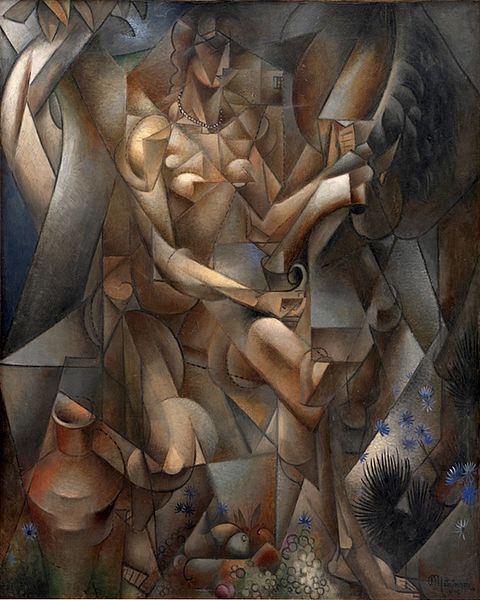This artwork features a modern, cubist-inspired painting composed of various geometric shapes like triangles, squares, and rectangles. The image centrally presents the figure of a woman, possibly sitting on a throne, with distinct elements that form a complex and intricate composition. Dominated by muted colors including blue, gray, tan, and occasional hints of red and black, the scene includes several discernible objects.

In the middle section, which is primarily brownish beige, the woman appears adorned with a necklace. Surrounding her are different items, such as vases and ceramic jugs, depicted at the bottom of the artwork. The edges of the painting are accented with gray and blue tones. Blue flowers and a black feather-like element also appear within the geometric structure.

Near the floor in front of the woman, a stuffed animal, possibly a rabbit, adds a touch of whimsy to the otherwise structured composition. The overall piece uses highlighted sections of white and darker shades to enhance the segmentation of shapes, contributing to the abstract yet somewhat identifiable representation of the woman and the surrounding objects.